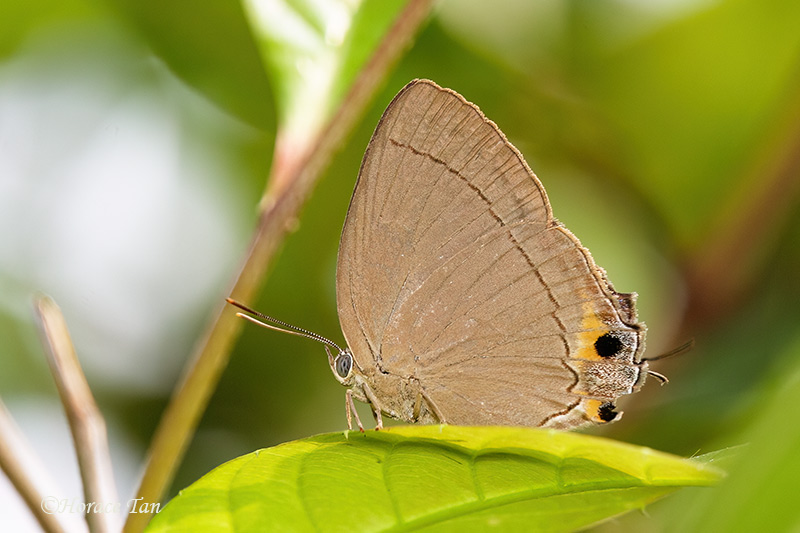This detailed photograph captures a side view of a tan-colored moth perched on a lime green leaf. Only one wing is visible, showcasing intricate details such as a light brown line running along the outer part, curving slightly at the bottom. Near this curve on the outer edge of the wing, there are two distinct yellow and black dots with a subtle grayish area beneath them. The moth's anatomy is partially visible, revealing four legs and a prominent gray eye, with two large antennae extending from the eye region. The moth stands on a leaf with a prominent stem leading to additional leaves, set against a blurred green and white background. Additionally, faint white text is inscribed in the image, potentially indicating the name of the photograph or the photographer, although it is hard to decipher.